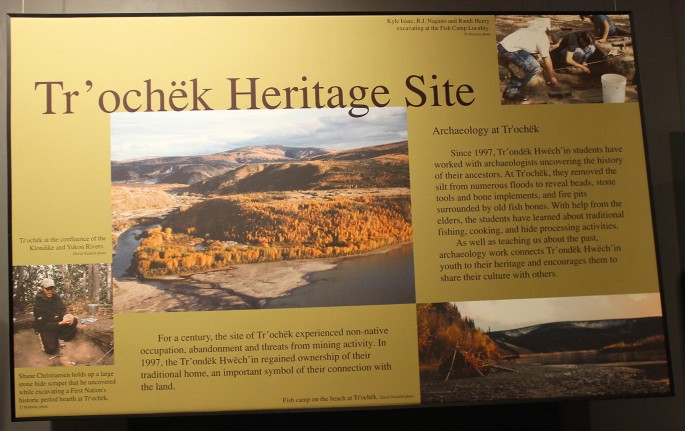This information placard for the Trochek Heritage Site, set against a gold background, provides a detailed glimpse into the site's historical and archaeological significance. The main title "Trochek Heritage Site" is prominently displayed in brown lettering. Below the title, a central image showcases a picturesque landscape featuring a striking blend of mountains, blue sky with clouds, and a patch of water surrounding an island densely populated with trees. To the left of this main image is a smaller picture of a person kneeling down, wearing a black sweatsuit and white cap, possibly engaged in some form of site investigation.

At the top corner of the placard, another image depicts individuals engaged in archaeological activities. A man in a white t-shirt and blue jeans is seen squatting, while another person, whose gender is indistinguishable, sits on the ground with a white bucket. The bottom of the placard features additional imagery of the heritage site, highlighting a scenic landscape with red, yellow, and brown leaves with mountains in the background.

Text on the placard details the site's significance, noting it has experienced non-native occupation, abandonment, and mining threats over the past century. In 1997, the Trochek people regained ownership of their traditional land, marking an important symbol of their enduring connection to the area. The placard also notes that since 1997, students have collaborated with archaeologists to uncover the site's rich history. Descriptive paragraphs elaborating on these themes further emphasize the site's historical and cultural importance.